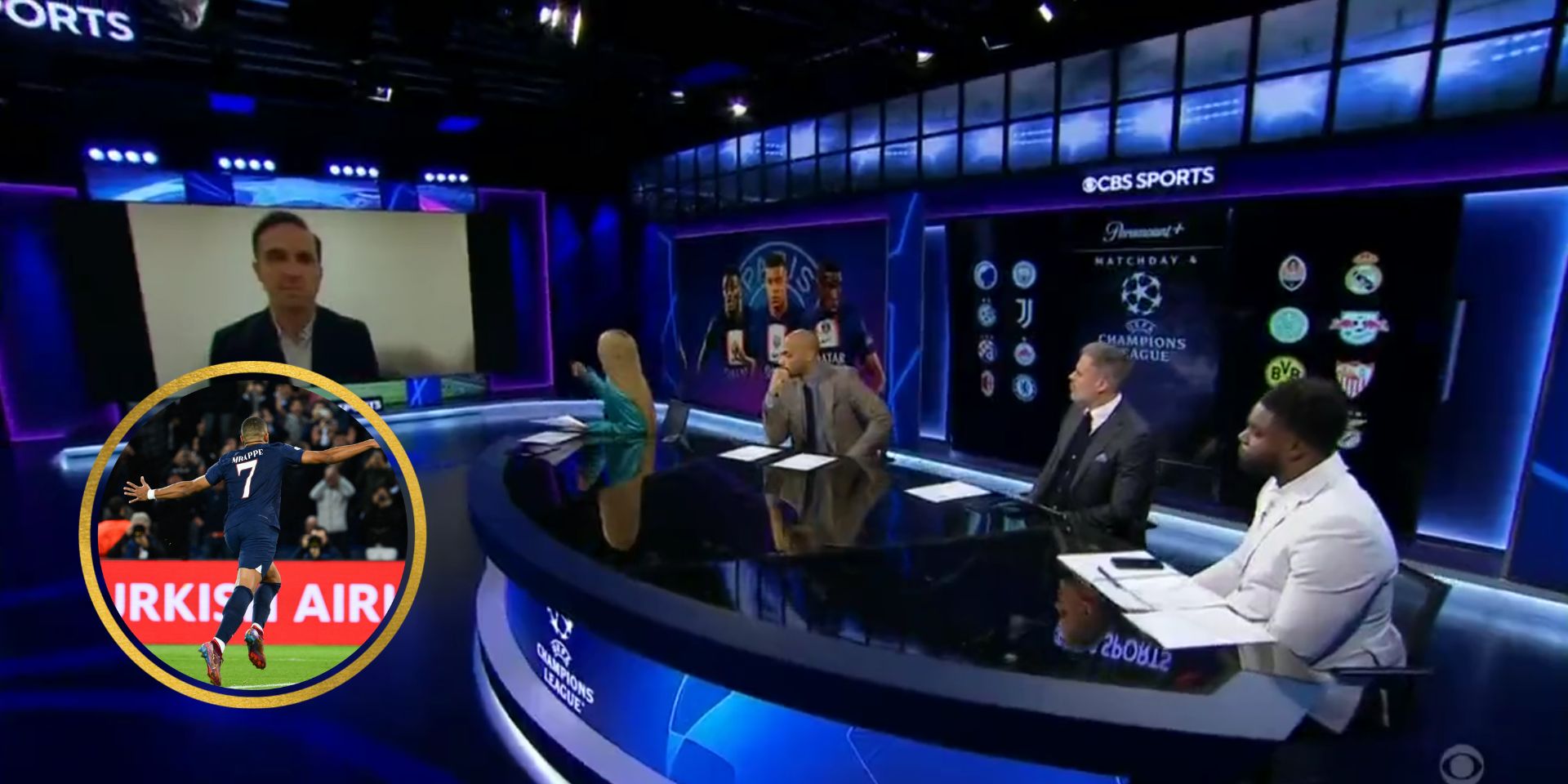This image captures a scene from a CBS Sports television show set, characterized by its predominantly blue background interspersed with white elements. A prominent row of blue rectangles spans from the top right corner towards the center. Below this pattern, "CBS Sports" is clearly displayed in white text. The set features a large glass-topped desk occupied by four sports reporters: a blonde woman, a bald black man, an older white man with gray hair, and a darker-skinned black man with hair. 

In front of each reporter, there are papers, and they are all dressed in suit jackets. Their attention is directed towards a monitor on the left side of the picture, which shows a man in a black coat and white shirt, possibly communicating with them via a video call. Positioned above the monitor are ceiling-mounted lights. Additionally, the left side of the screen features a circular inset image of the soccer player Mbappe, wearing the number seven in a blue jersey, running on a green pitch with his arms extended in celebration. Just behind him, there's a barrier with "Turkish Air" written in white letters on a red background.